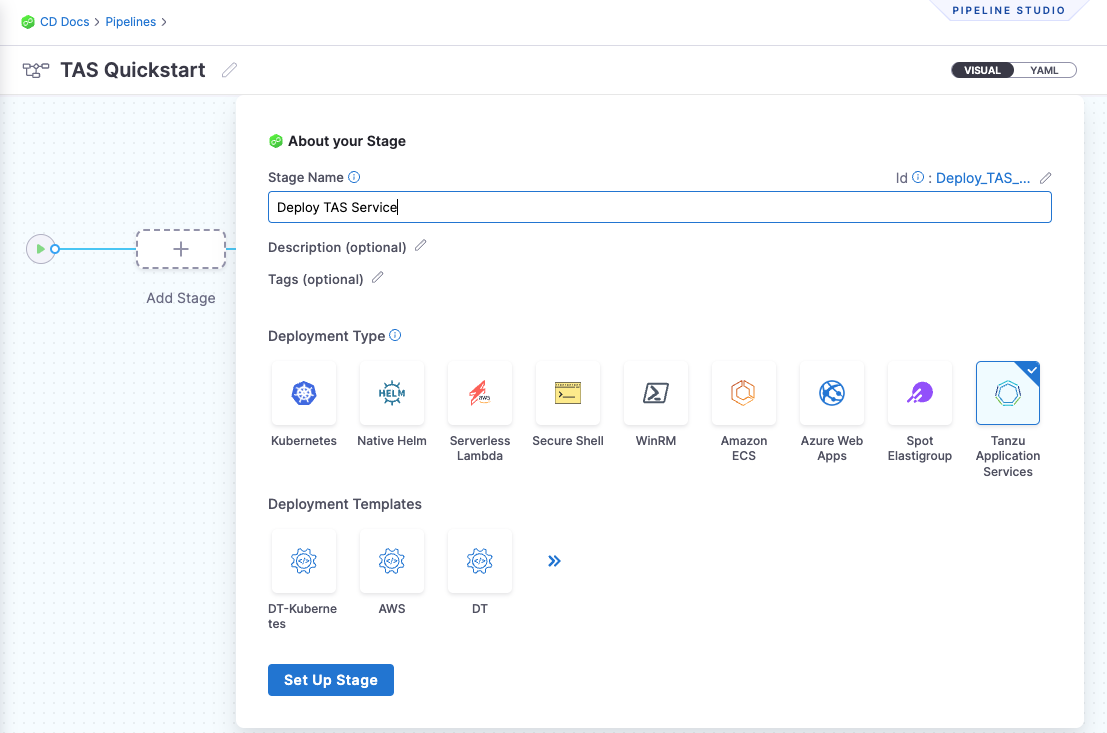This screenshot captures the interface of a program or webpage titled "Pipeline Studio," identifiable by its name displayed in blue text at the top right, adjacent to a trapezoid-shaped logo. The interface belongs to a section categorized under "Pipelines," with a navigation path visible in the top left corner starting from "CD Docs" and leading to "Pipelines." 

In the top left corner, there is a note labelled "TAS Quick Start." The central part of the interface presents detailed information about a specific stage in the pipeline termed "Deploy TAS Service." 

The title "About Your Stage" introduces this section. Below it, various fields are presented:
- **Stage Name:** "Deploy TAS Service"
- **Description (Optional):** Currently blank.
- **Tags (Optional):** Currently blank.
- **Deployment Type:** "Tanzu Application Services" is selected from multiple options.
- **Deployment Templates:** No template has been selected.

At the bottom of this interface, a prominent blue button labeled "Setup Stage" is available for further configuration.

The overall design is clean, with a clear structure guiding the user through the various stages of setting up a pipeline.